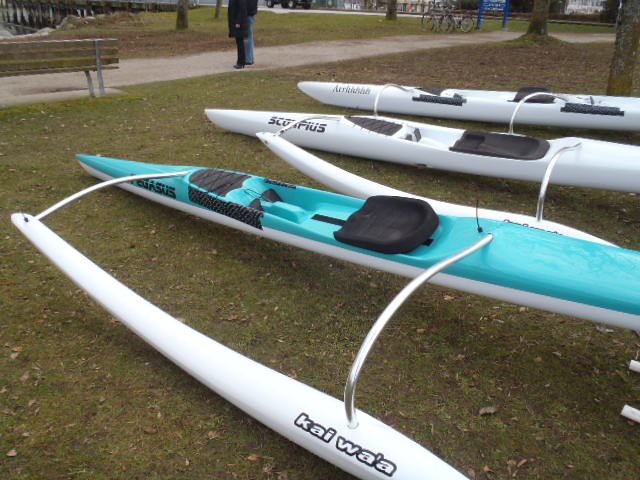In a vibrant park setting during late autumn or early winter, three personal sea kayaks rest on the sparsely grassed, somewhat brown ground. The kayaks stand near a paved path, beside which the bottom halves of a couple can be seen. One striking aqua-colored kayak in the center is equipped with a white stabilizing bar akin to those seen on Hobie sailboats; it features a black seat and is marked with the name "Kai Wai." Flanking it are two solid white kayaks, each also equipped with black seats, though they appear to be of different brands. In addition to these single-person kayaks, the park scene includes parked bicycles, a nearby waterway hinted at in the corner, several tree trunks anchoring the landscape, and a park bench that highlights the tranquility of the setting.